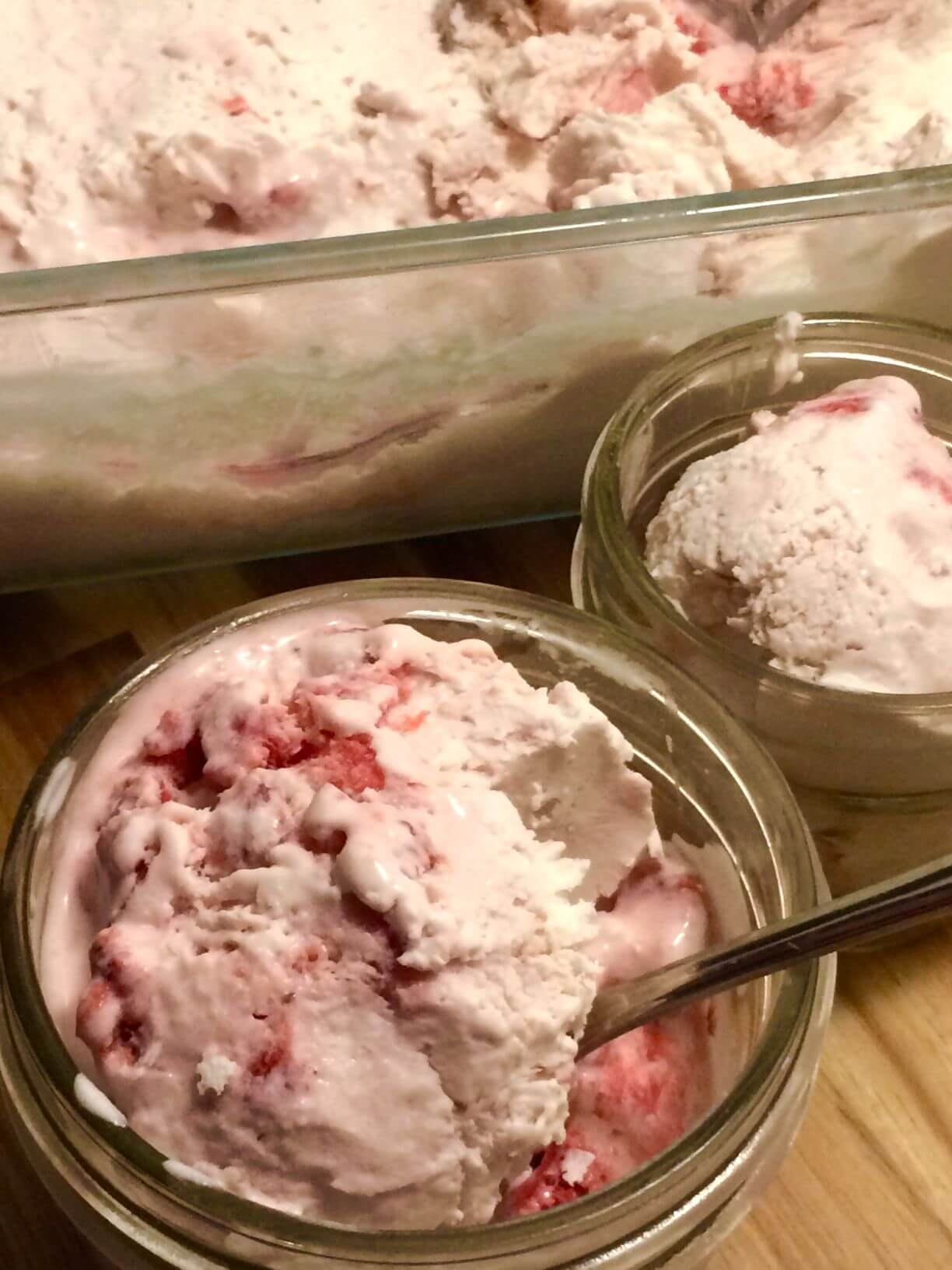This rectangular photograph showcases a delightful display of strawberry ice cream, resting on a brown wooden table. The image features three clear containers: two smaller glass bowls in the foreground and a larger, obscured serving dish in the background. The ice cream in the glass bowls is a pleasant pink hue, speckled with bits of strawberry. In the foremost bowl, a spoon is placed at an angle, partially submerged in the ice cream and resting on the bowl’s edge. Behind this, another glass bowl holds similarly appealing strawberry ice cream, though it appears slightly fresher and less melted. Occupying the top portion of the image is a long, partially visible serving dish or tub, filled with more of the same delectable ice cream, creating an impression of homemade preparation and serving. The entire setup, with the table visible beneath, conjures a sense of a cozy gathering, perhaps in a home or an inviting ice cream shop.